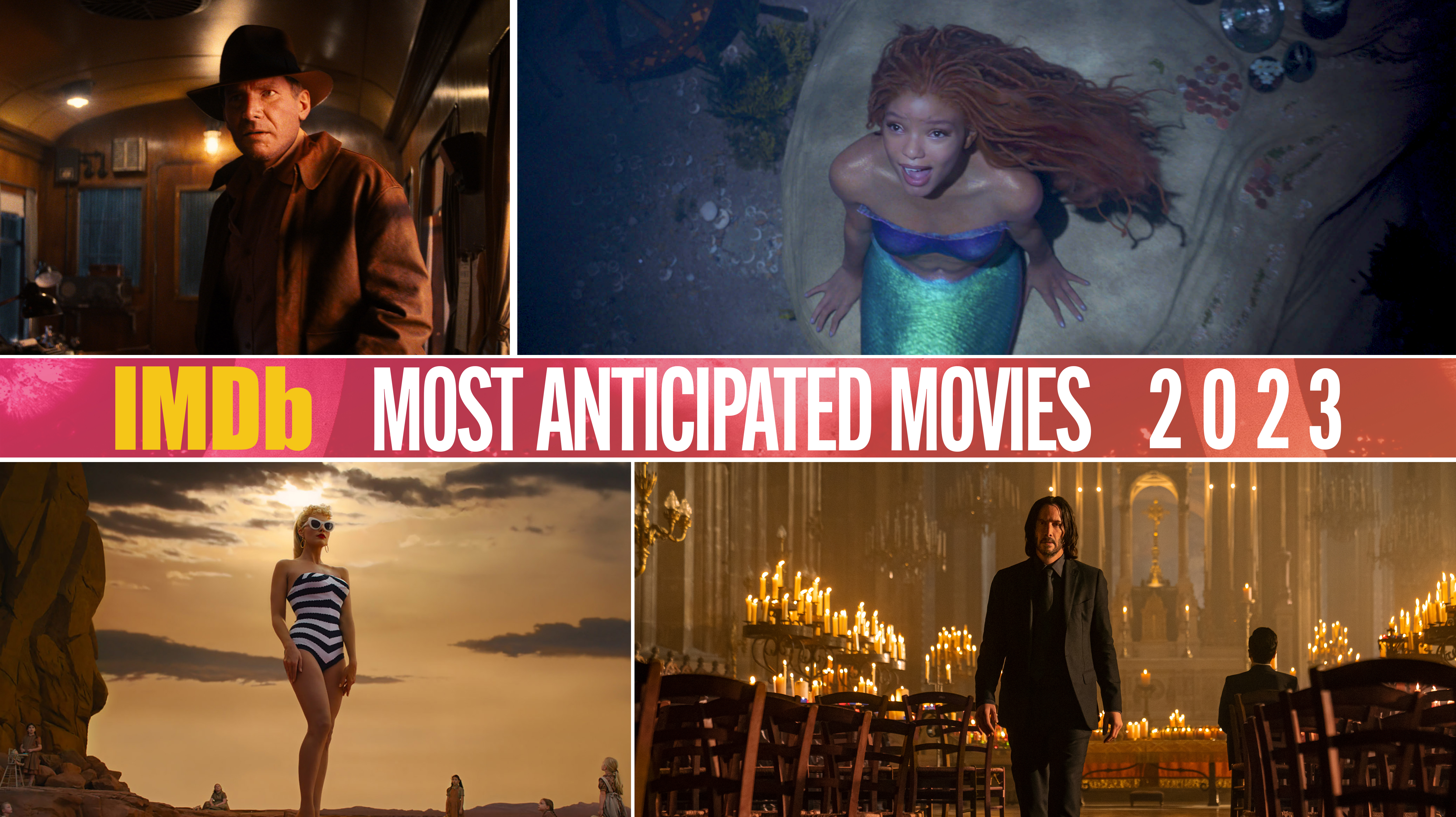This image features a collage of four movie stills with a reddish-orange horizontal banner in the center that reads "IMDb Internet Movie Database" in yellow letters and "Most Anticipated Movies 2023" in white. In the top left, Harrison Ford portrays Indiana Jones, dressed in a tan jacket and brown hat, set in a location resembling a train car or rounded roof structure. The top right highlights a modern rendition of The Little Mermaid, with a Black mermaid character in a turquoise tail and blue bikini top, sitting on a large gray stone and singing underwater. The bottom left showcases Barbie in a black and white striped swimsuit and sunglasses, posed in an outdoor scene with rocks and sky. In the bottom right, Keanu Reeves stars as John Wick, donning an all-black suit and walking through a candle-lit cathedral filled with chairs and tables.